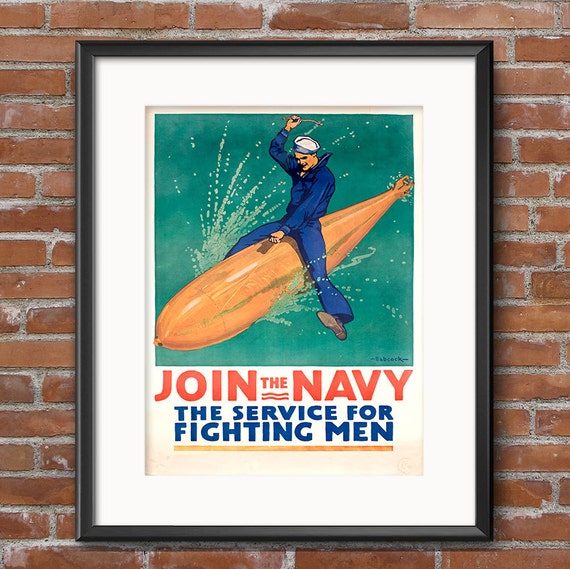A photograph captures a beautifully framed vintage Navy advertisement mounted on an industrial-style brick wall in a restaurant or similar warehouse-like setting. The wall features brown bricks with gray mortar, perfectly complementing the black frame and its inner white border. The framed advertisement depicts a sailor in a traditional blue uniform and white hat, riding an orange torpedo with a dynamic, rodeo-like flair—his right hand gripping the torpedo while his left hand is raised, mimicking a bull rider. Throughout the image, shades of blue represent the water splashing around him. Boldly at the bottom, the text "Join the Navy" appears in red, underlined in gold, followed by "the service for fighting men" in blue.